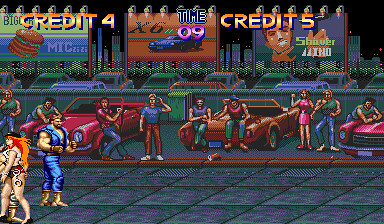This image is a vivid screenshot from an unspecified video game, depicting a landscape-oriented scene. At the very top, there's a series of brightly colored texts: "Credit 4" and "Credit 5" are displayed in a blend of orange and yellow, bordered with blue. Dominating the upper center is the word "TIME" written in blue, followed directly beneath by "09" in striking pink.

In the game environment behind these texts, three distinctive billboards capture attention. The first billboard displays the word "BIG" alongside an image of a cheeseburger, with the letters "M-I-C-Z-Z-I-Z-I" visible. The adjacent billboard features the text "X6" with an illustration of a car beneath it. The third billboard showcases an individual shaving, accompanied by the word "SHAVER" and the letters "I-N-O."

Below these billboards, a row of cars stretches from left to right, further grounded by a fence. Leaning against these cars are various people, creating a lively scene. At the very bottom of the image, from the left to the right, there’s a pattern of slates marked with X's in a shade of dark blue-green. On the bottom left, individuals with orange hair and clad in blue outfits add a dynamic element as they walk around the area.